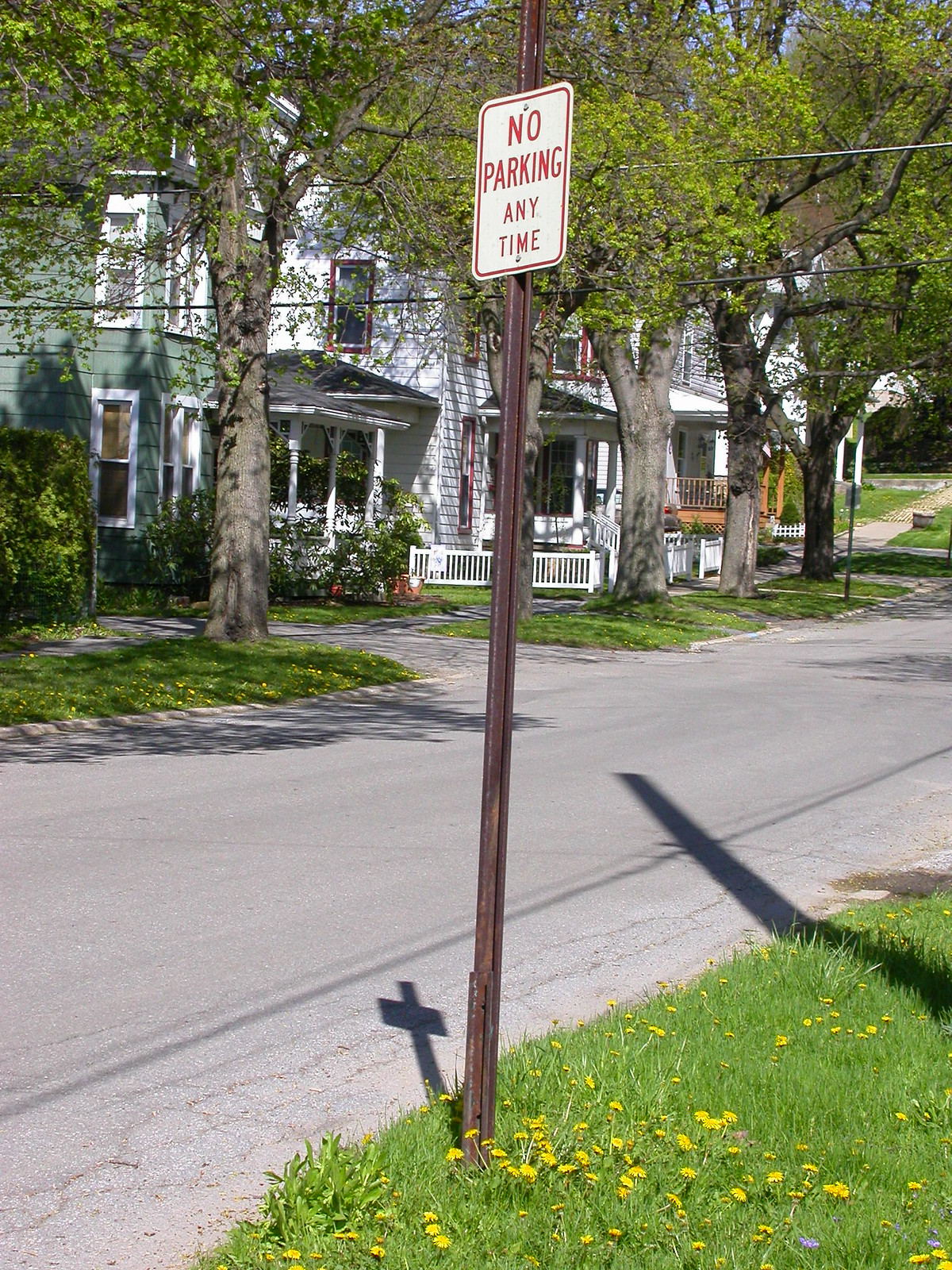This photograph captures a quiet residential street bordered by light gray asphalt with noticeable cracks along the edges. In the bottom right corner, a patch of green grass is dotted with cheerful yellow dandelions. Nearby, a "No Parking Anytime" sign, marked by its white face and red border, stands tall on a rusty metal post. On the left side of the street, another grassy area leads up to trees with rough brown bark and lush green leaves. A charming home with pristine white siding and a green roof sits prominently to the left, while further down the street, another house with a welcoming front wooden deck comes into view, adding to the cozy neighborhood ambiance.